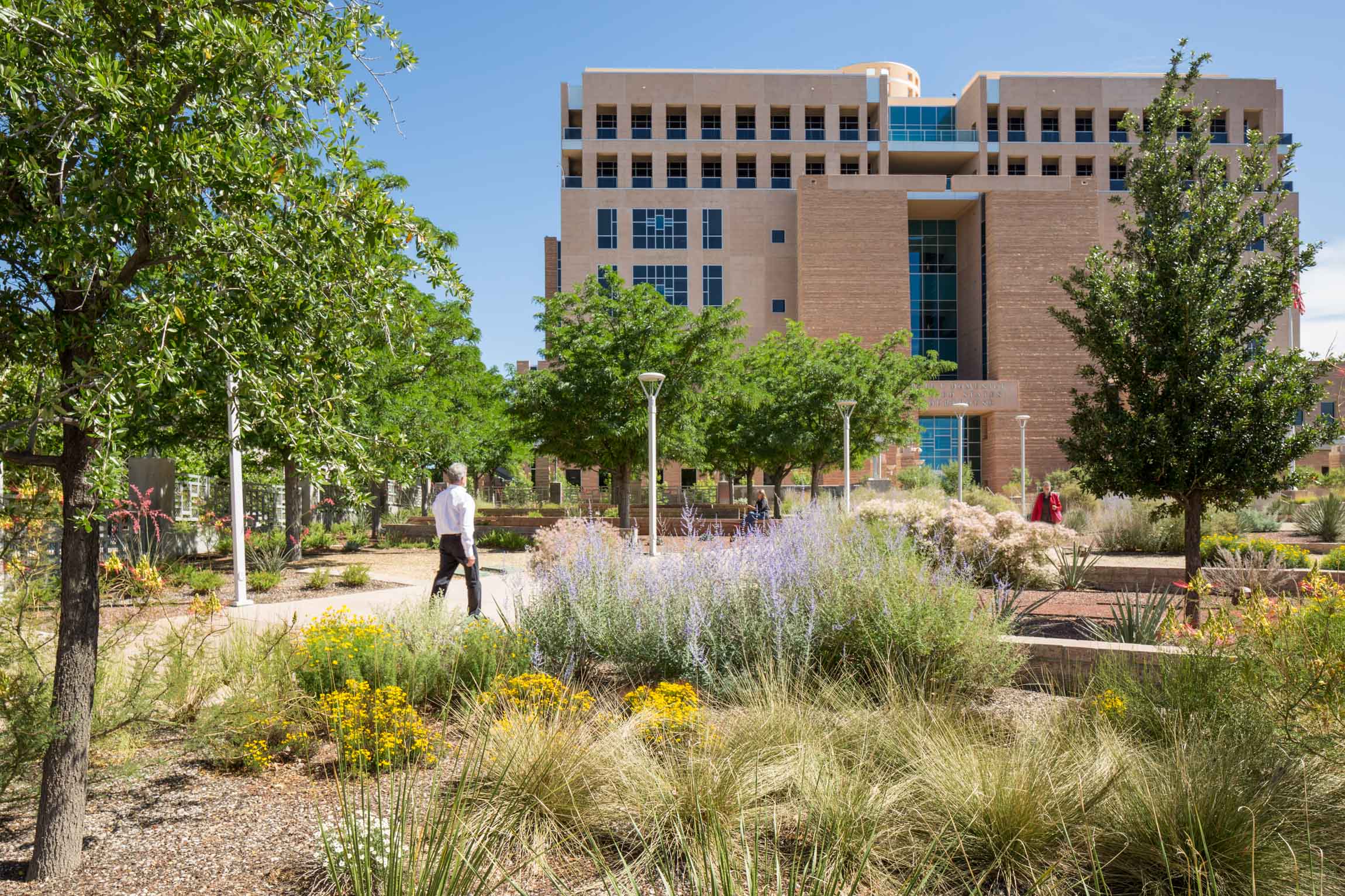The image depicts a serene afternoon scene on a southwestern college campus, characterized by a tan adobe-colored building approximately ten stories high. The building, off-centered to the right, exhibits a modern design with a series of small windows near the top and larger windows down the side, culminating into a cluster of small square windows at the entrance. The grounds feature water-conscious landscaping with dry brush, desert plants, a variety of shrubs, and strategically placed rocks, reflecting the arid climate.

In the immediate foreground, there are two trees, one on the left and one on the right. A well-maintained pathway, bordered by five visible overhead streetlights, leads towards the building. A man with gray hair, dressed in a white shirt and black pants, is seen walking on the pathway towards the structure. He is positioned slightly to the left. Walking in the opposite direction, towards the camera, is an unidentified individual in a red jacket, making it difficult to ascertain their gender due to the distance. Additionally, further down the pathway, a woman with blonde hair, wearing a black top, appears to be gazing at the surrounding trees, adding to the tranquil ambiance of the campus.